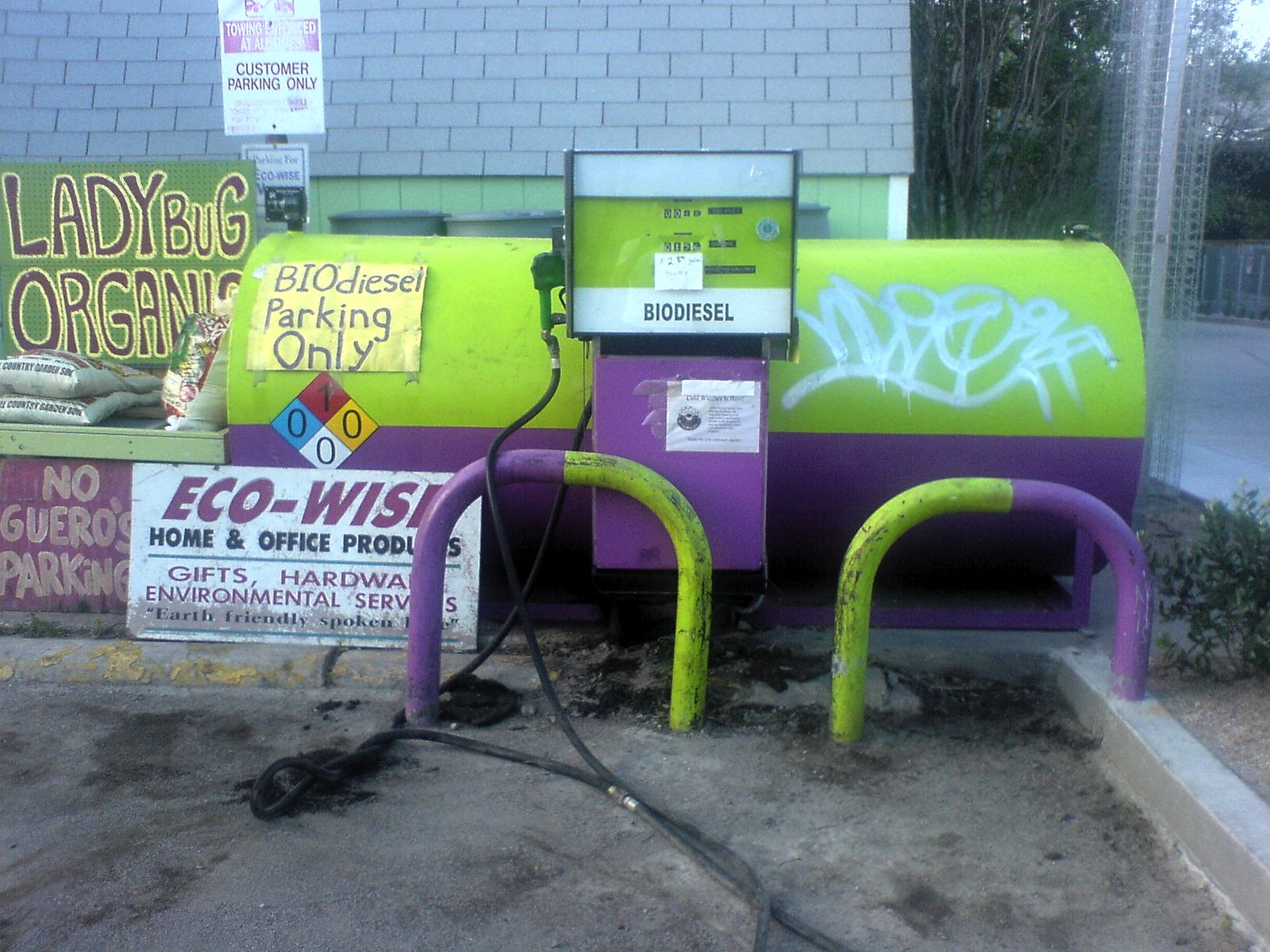In this vibrant outdoor scene, a lime green and purple biodiesel tank is prominently featured, complete with coordinating green and purple pump hoses lying on the ground. A sign on the left side of the tank reads "biodiesel parking only" in black text on a yellow background, while a smaller sign with the purple text "EcoWise, home and office products, gifts, hardware, environmental services, earth friendly spoken here" rests on the concrete below. Nearby, another handwritten sign with a green background states "ladybug organics," above bags stacked on a shelf and a table, with a "no garros parking" sign below. In the background, a little shed can be seen behind the tank, while the right side of the image reveals a curb, some bushes, and a line of trees.